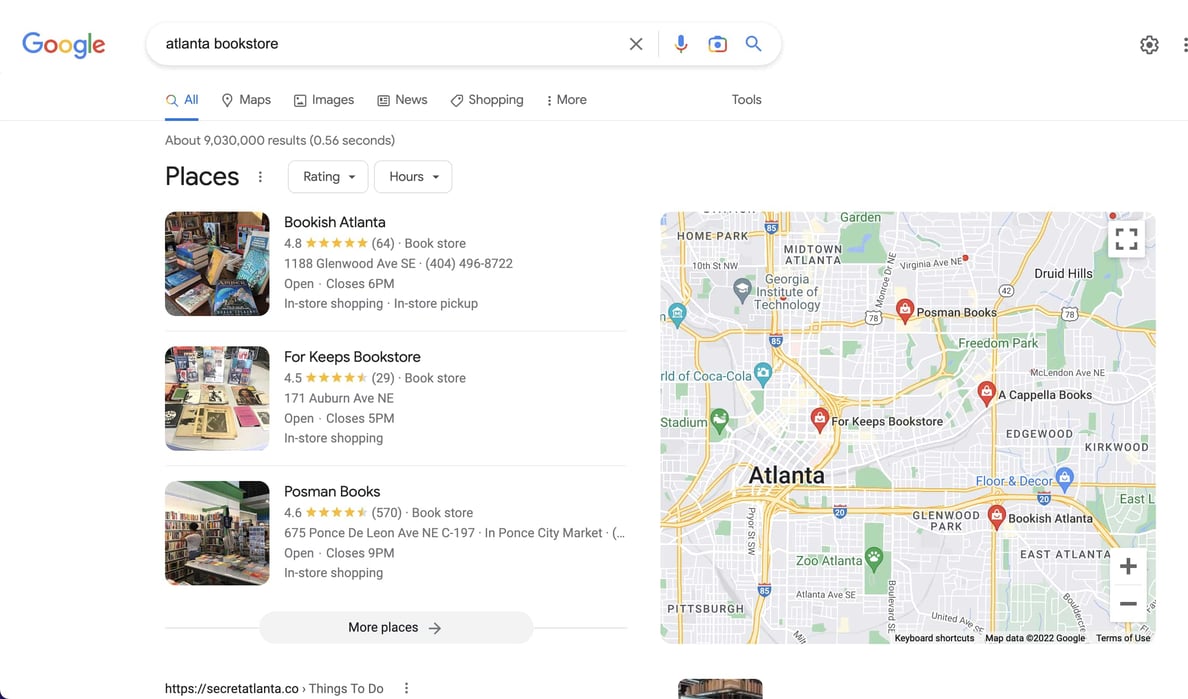The image is a detailed snapshot of a Google search results page focused on the query "Atlanta bookstore." The right-hand side features a map of Atlanta, pinpointing the locations of various bookstores, including Bookish Atlanta, For Keeps Bookstore, and Posman Books. Additionally, landmarks such as Zoo Atlanta, a stadium, and the Georgia Institute of Technology are also marked.

On the left side, a series of images depict different books in varying orientations—some standing, some lying on a wooden surface—with covers in diverse colors like blue, white, black, yellow, orange, brown, and turquoise, though the text on the book covers is too small to read.

Detailed information is provided for each bookstore:

- **Bookish Atlanta**: Rated 4.8 stars based on 64 reviews, located at 1188 Glenwood Ave SE. The bookstore offers in-store shopping and pickup, and is open until 6 PM. Contact number: 404-496-8722.
- **For Keeps Bookstore**: Rated 4.5 stars based on 29 reviews, located at 171 Auburn Ave NE. It also offers in-store shopping and remains open until 5 PM.
- **Posman Books**: Situated at 675 Ponce de Leon Ave NE, within Ponce City Market (Suite C-197), this bookstore offers in-store shopping and is open until 9 PM.

Below this information, there are additional places listed, along with clickable links for more details and activities to do in Atlanta. The caption provides a comprehensive overview of the search result page, including both visual elements and textual data.